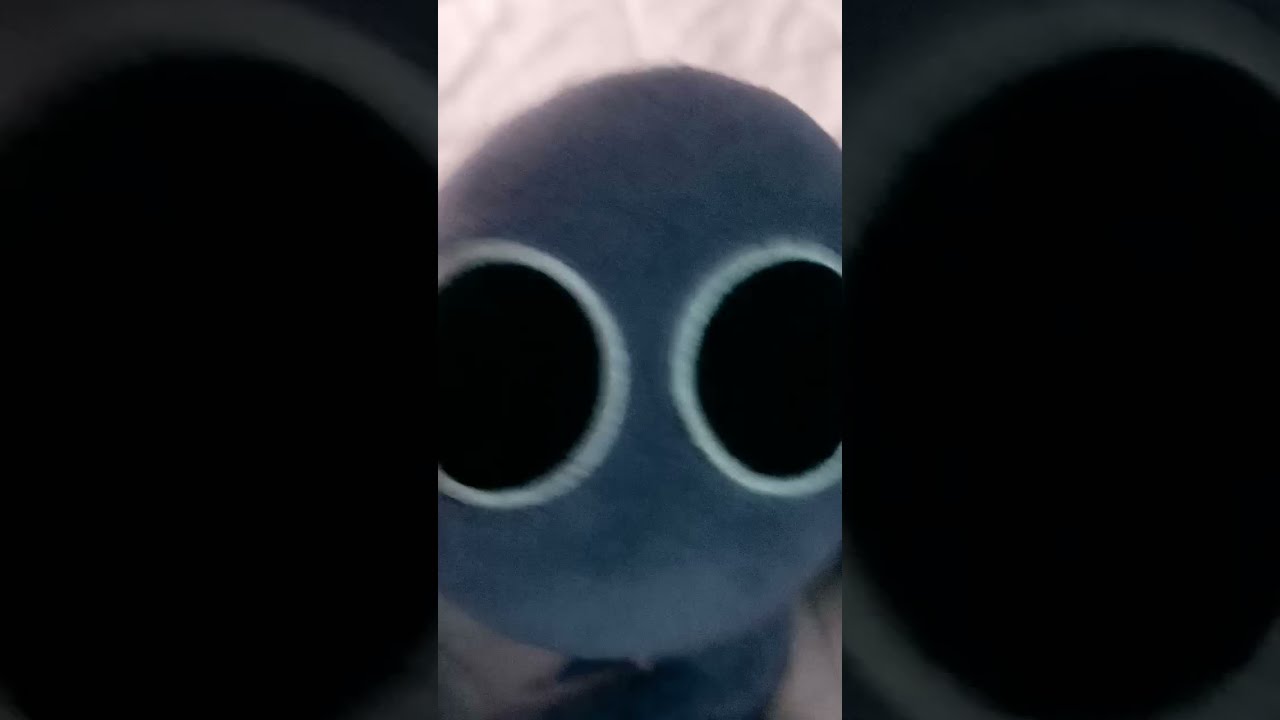The image features a slightly blurry photograph that appears to be taken with a cell phone. It's divided into three landscape-oriented panels with the left and right panels being black and opaque, which serve to emphasize the center panel. The central focus is a grayish-blue soft, fabric-like circular object, resembling a felt or micro-suede texture. This object is adorned with two large black circles with white borders, positioned in a way that evokes the appearance of eyes on a creature or character. The background consists of a blurry off-white surface, possibly white bedsheets. The object resembles a large round blue felt ball, devoid of any discernible facial features such as a nose or mouth. The overall image composition and texture give the impression of a plush toy or fabric-based art piece.